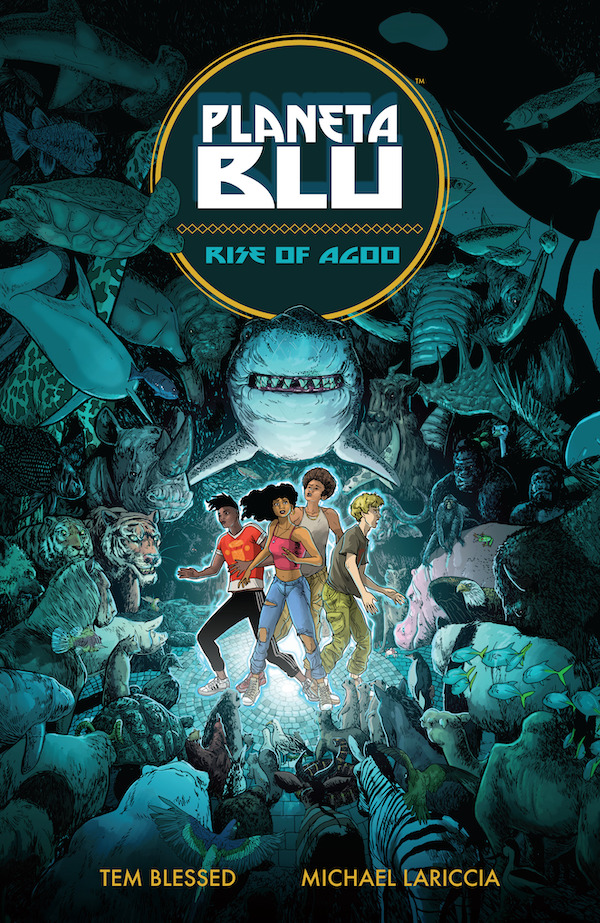This is an intricately detailed cover of a book, possibly titled "Planeta Blu: Rise of a God," showcasing a vibrant and dynamic digital illustration. The background features a gradient of lighter blues, teals, and turquoise hues, filled with a plethora of animals, such as turtles, mammoths, gorillas, tigers, hippos, zebras, and various fish, arranged to encircle the central characters. Amidst this teal-toned backdrop, the middle of the cover bursts into a more vivid array of colors, highlighting four teenagers, three African American and one white, seemingly embarking on a quest inside what appears to be a cave. The girl in the middle sports a pink top and long black hair, flanked by a boy with black hair in a red shirt on her left and another boy with blonde hair wearing a brown shirt on her right. Above them looms a shark, its teeth front-facing, almost as if it's protecting the teens. The title "PLANETA BLU" is emblazoned in white letters within a gold circle at the top, with "RISE OF A GOD" in teal beneath it. The creators' names, Tim Blessed and Michael Laricia, are printed in yellow at the bottom left and right corners, respectively. The combination of animated characters and a multitude of animals creates an engaging and adventurous scene, making the teenagers the vibrant focal point amidst a captivating array of wildlife.